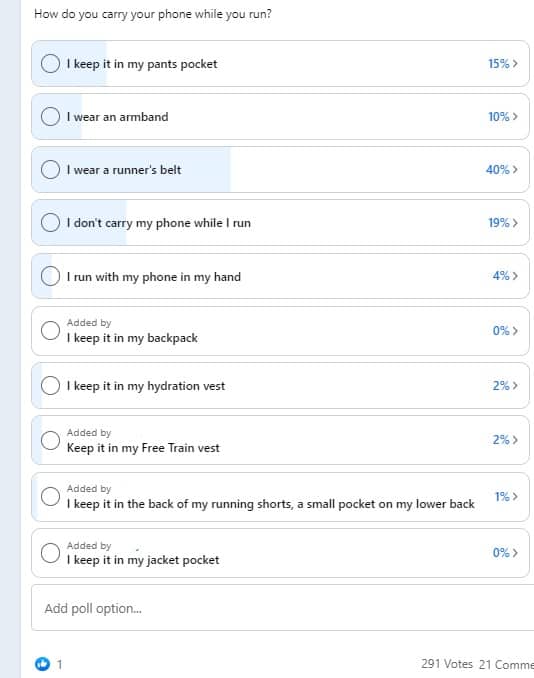The image depicts a poll titled "How do you carry your phone while you run?" at the top. It features 10 detailed options for respondents to choose from, along with the corresponding percentages for each option, prominently displayed on the right side. Here's a breakdown of the results:

1. **I keep it in my pants pockets:** 15%
2. **I wear an armband:** 10%
3. **I wear a runner’s belt:** 40% (highest percentage)
4. **I don’t carry my phone when I run:** 19%
5. **I run with my phone in my hand:** 4%
6. **I keep it in my backpack:** 0%
7. **I keep it in my hydration vest:** 2%
8. **I keep it in my FreeTrain vest:** 2%
9. **I keep it in the back pocket of my running shorts:** 1%
10. **I keep it in my jacket pocket:** 0%

The bottom right of the image notes that there are 91 votes and 21 comments on the poll. The bottom left features a blue 'like' button with one like indicated. There is also an option at the bottom of the poll to "Add a poll option" for additional input. The percentage of responses for each option is highlighted with a blue outline to visualize the distribution of choices.